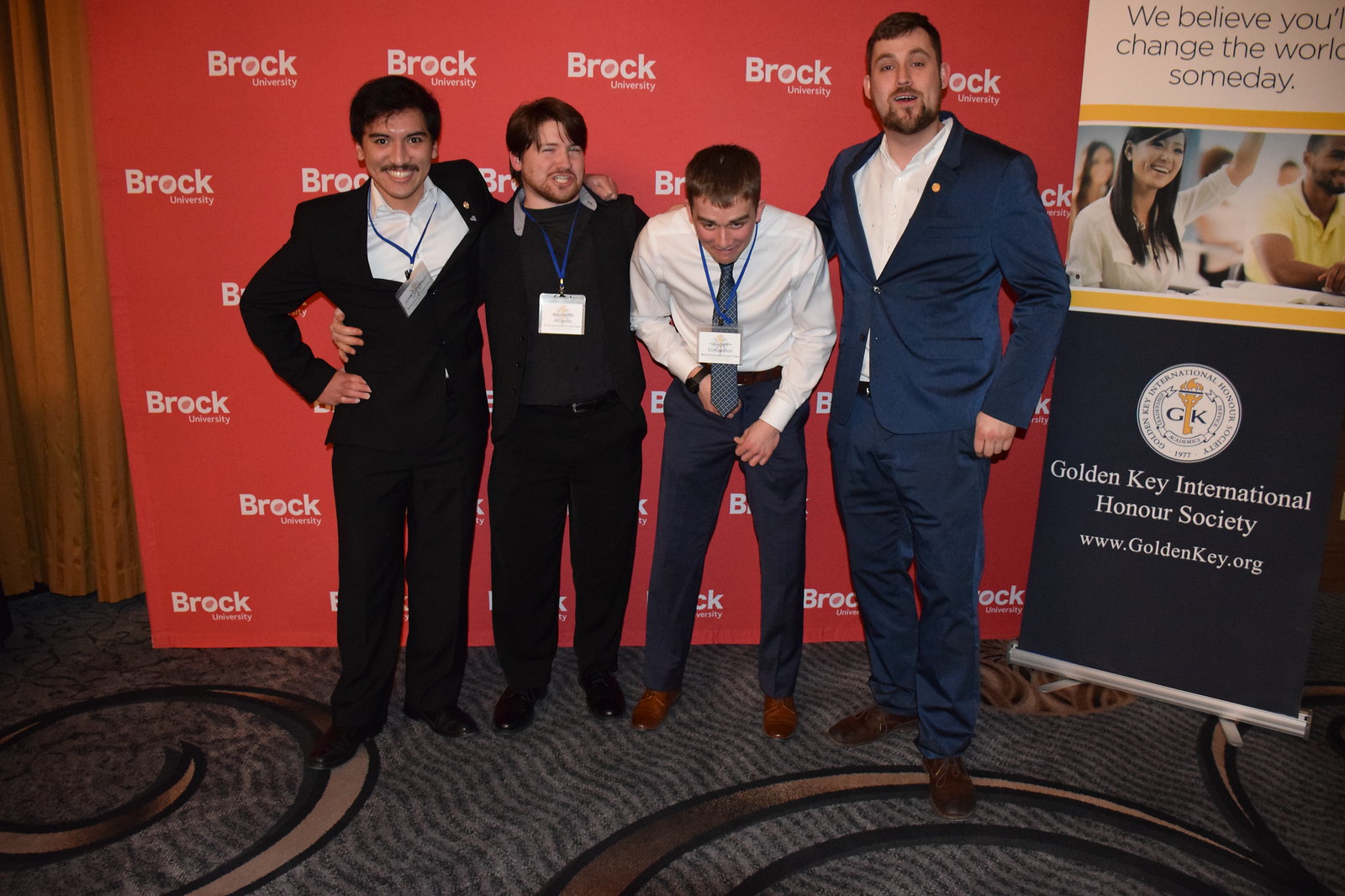In the center of this indoor image, four well-dressed men stand directly facing the camera, all wearing suits. The man on the far right is in a blue suit and pants with a dress shirt, while the man on the left wears a white shirt and tie with dress pants. The two men in the middle sport black shirts and black pants, with one of them having a black t-shirt underneath his blazer. Behind these individuals is a prominent sign that reads "Brock University" repeatedly in an orange-ish tone. To their right, another sign, featuring an image of people raising their hands in a classroom, reads "We believe you'll change the world someday," with "Golden Key International Honor Society" written below it along with their website, www.goldenkey.org. A golden key symbol, flanked by the letters GK and a laurel, adorns the sign. The multi-color, multi-textured carpet on the ground adds to the vibrant setting of this picture taken in what appears to be a college environment. The men, who seem to be of mixed races, are impeccably dressed in dark-colored slacks, enhancing the formal ambiance of the scene.